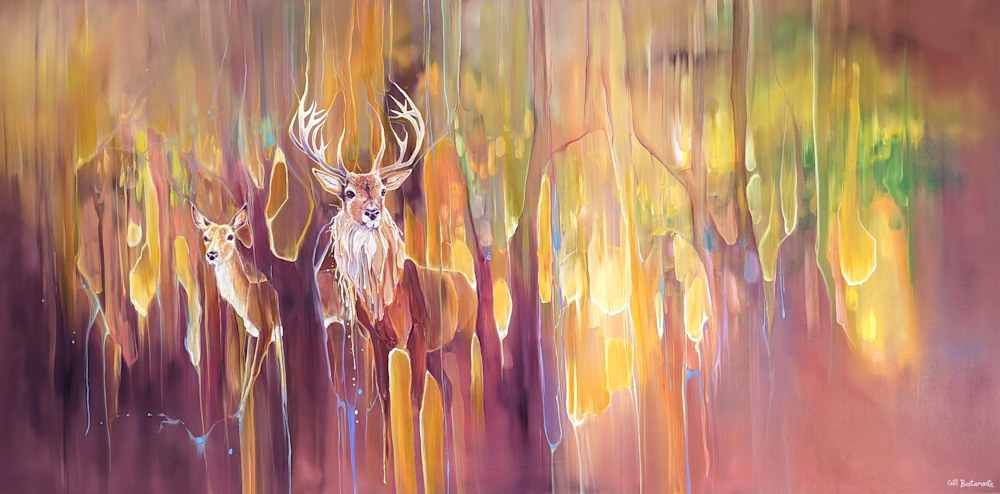This vibrant watercolor painting features two light brown deer set against a striking, multi-colored background. The larger male deer, located near the center-left of the image, is distinguished by its grand white antlers and white fur trim around its neck, with black eyes adding a stark contrast. To the left of this deer, a smaller doe or fawn, lacking antlers, is partially obscured, blending beautifully with the background yet still noticeable by her delicate brown body and legs. The scene appears to hover in a space adorned with an array of vertical color streaks in purples, blues, pinks, yellows, and greens, creating an impression of dripping paint that flows into a darker purple area in the bottom left corner. The background intensifies in brightness towards the center, enhancing the painting's lively and dynamic effect. Amidst these colors, subtle shapes reminiscent of trees add depth to the scene. The artist’s signature, though small and illegible, is positioned in the lower right corner, marking this as a captivating and vibrant piece of art.